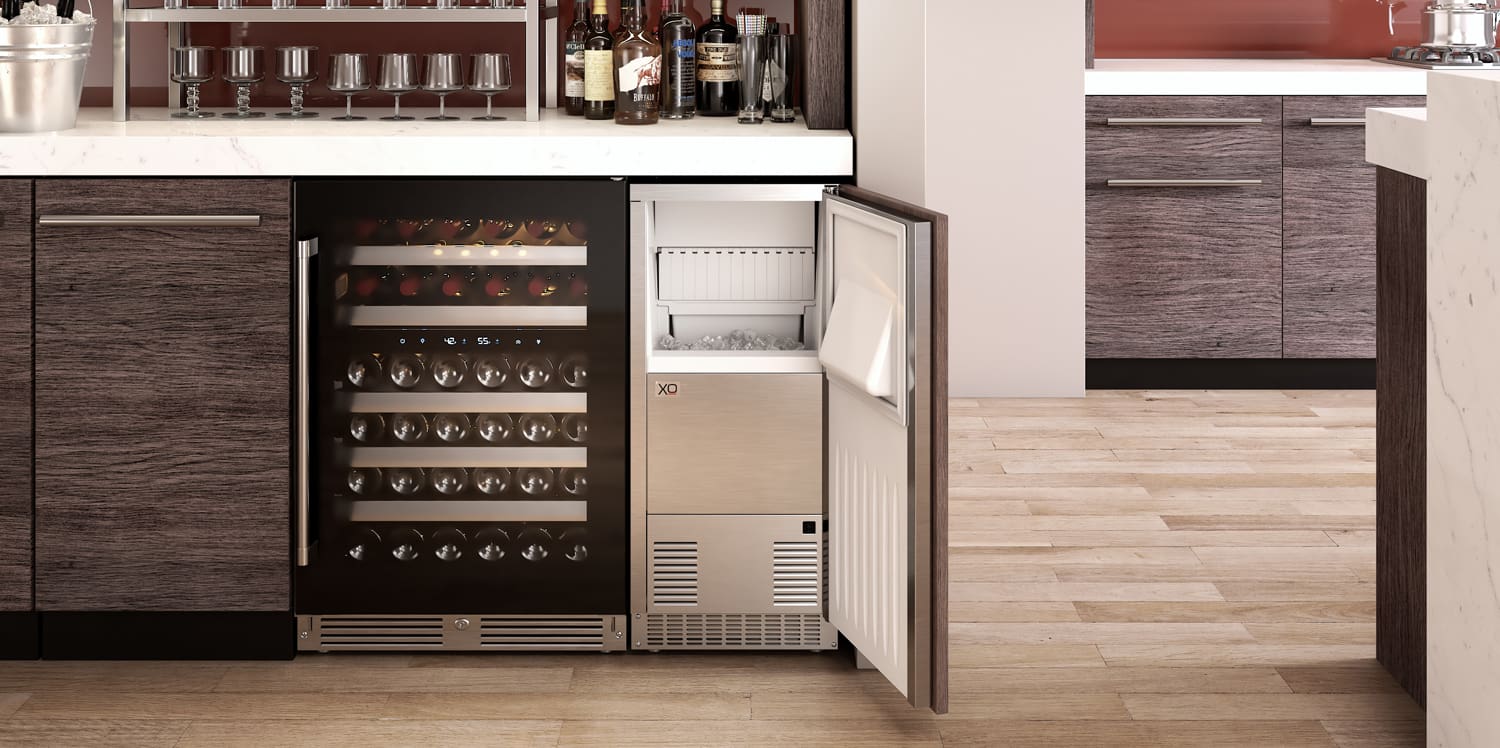The photograph appears to be a staged, stock photo showcasing a stylish drink station, possibly in a remodeled kitchen or a butler's pantry, often found in homes or hotels. The focal point is an open ice chest, built into the sleek, modern brown cabinetry underneath the white marble countertop. Adjacent to the ice chest is a wine fridge of matching size and design. The countertop is adorned with a variety of liquor bottles, all clearly labeled, and a silver ice bucket filled with ice. Several metal cups and measuring cups are also present, enhancing the bar setup. The floor features beige and dark brown alternating wood panels, possibly pine hardwood, adding a rustic charm. The walls, painted in a maroon hue, contrast starkly with the clean, modern fixtures, contributing to the image's sophisticated yet cozy ambiance.